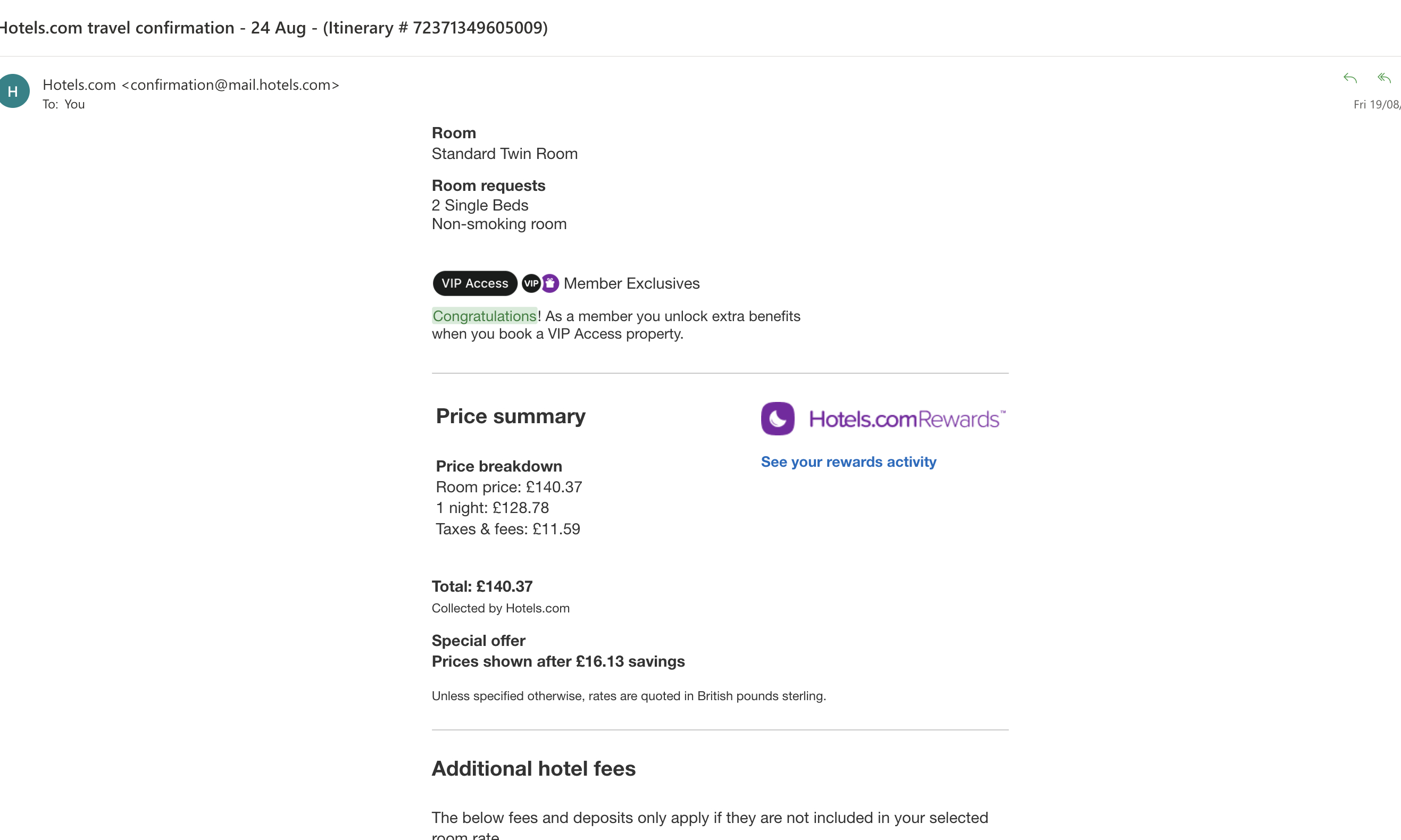**Detailed Caption for Hotels.com Travel Confirmation Screenshot:**

This image is a detailed screenshot of a travel confirmation email from Hotels.com, dated August 24th. The email, sent from Hotels.com confirmation at mail.hotel.com, is displayed on a white background with black text. It pertains to a hotel reservation with the following specifics:

- **Room Details**: Standard Twin Room with two single beds, non-smoking.
- **VIP Access**: Indicated by the label "VIP Access, Members Exclusive", with a green marker highlighting the text "Congratulations! As a member, you unlock extra benefits when you book a VIP Access property."

**Price Summary**:
- Room cost: £140 (or €140, currency not explicitly stated).
- Breakdown: One night rate is £128, with taxes and fees amounting to £11.59, making the total £140.37.
- Annotations include: "Price is shown after £16.13 savings," with mention that rates are quoted in British pounds sterling unless specified otherwise. Additional hotel fees may apply if not included in the room rate.

Finally, Hotels.com Rewards is displayed in purple with a moon icon.